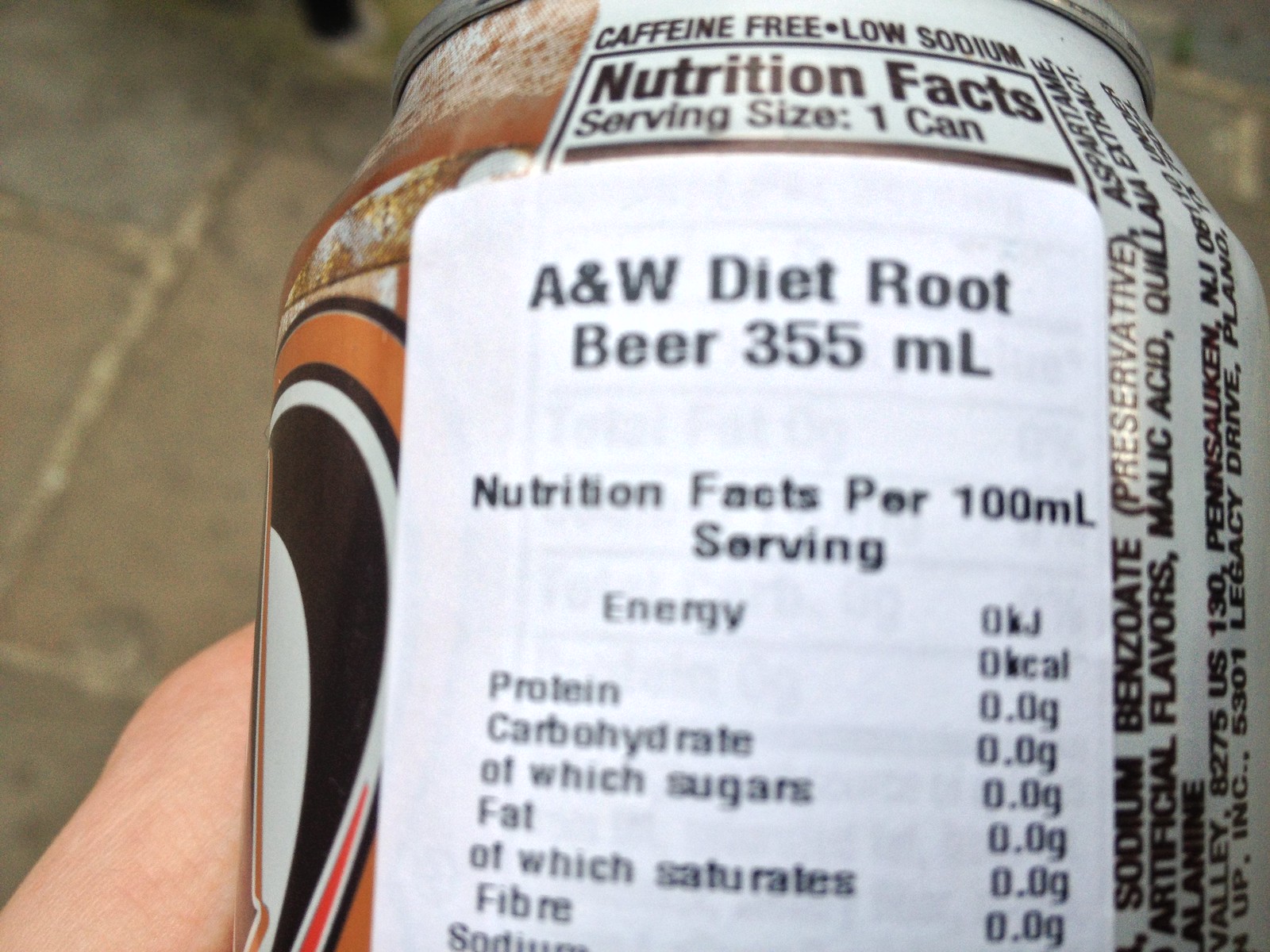This image features a close-up of a can of A&W Diet Root Beer positioned prominently in the foreground. The can is shown from its upper half, with the first half of its label clearly visible on the left-hand side. The distinctive branding includes a brown background typical of root beer packaging and an orange, white, and black striped logo beneath it. The rest of the can's label primarily consists of nutrition facts, though they're obscured by a white label affixed over the original. This label reads: "A&W Diet Root Beer, 355 mL." It further details the nutritional information per 100 mL serving, indicating that the values for energy, protein, carbohydrate, sugars, fat, saturates, and fiber are all zero.

In the blurry background, a stone pathway is partially visible. An obscured hand, showing just the side without any fingers, can be seen near the can, adding a touch of human presence to the scene. The overall composition highlights the can while providing context through the soft-focus background elements.